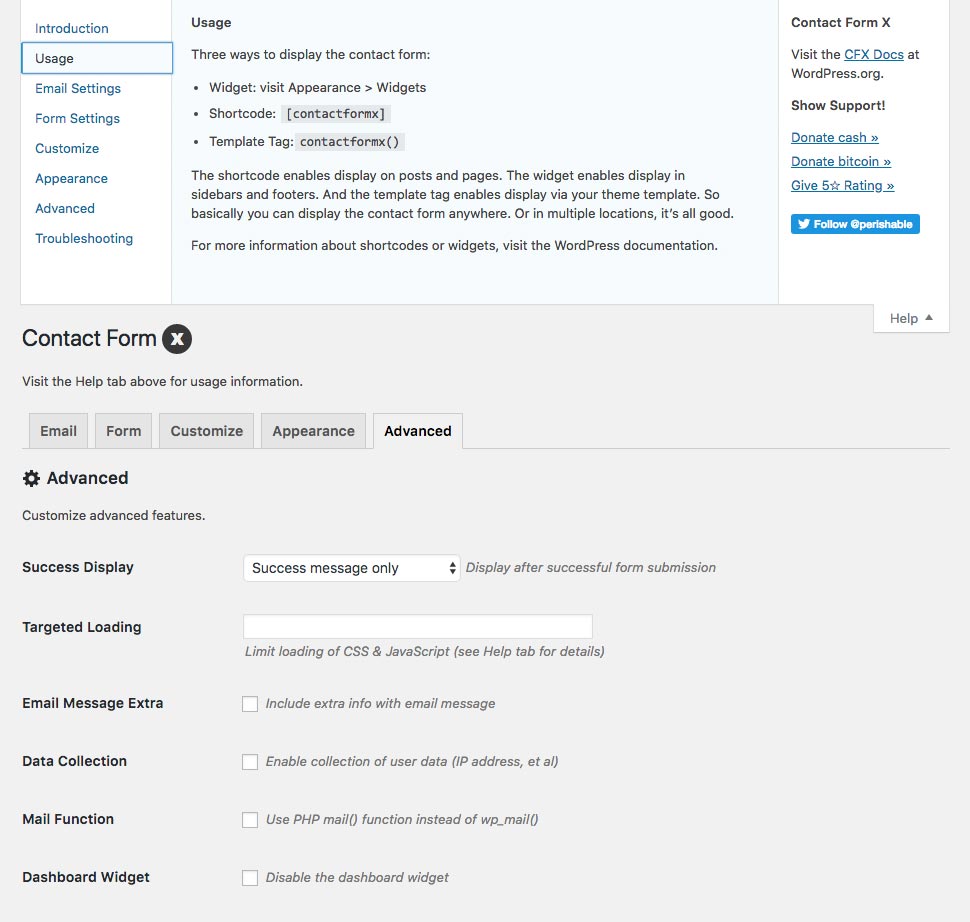Here is a detailed and cleaned-up caption:

---

The image displays a WordPress contact form interface. On the left, there is a left-justified navigation bar that includes the following options in a list: Introduction, Usage, Email Settings, Form Settings, Customize Appearance, Advanced, and Troubleshooting. The 'Usage' section is currently selected. On the right side, detailed information about displaying the contact form is presented. It outlines three methods to display the contact form:
1. **Widget**: Accessible via Appearance > Widgets.
2. **Shortcode**: Use `[contact_form_x]` to insert within posts and pages.
3. **Template Tag**: Utilize `<?php contact_form_x(); ?>` to incorporate it directly into theme templates.

Each method allows placement in various locations such as sidebars, footers, or any section of a page. Additional pointers direct users to WordPress documentation for more information about shortcodes and widgets. The bottom section provides links for user support including options to donate cash, donate Bitcoin, give five-star ratings, and follow on Twitter. Below this, a sample of the Contact Form X is showcased.

---